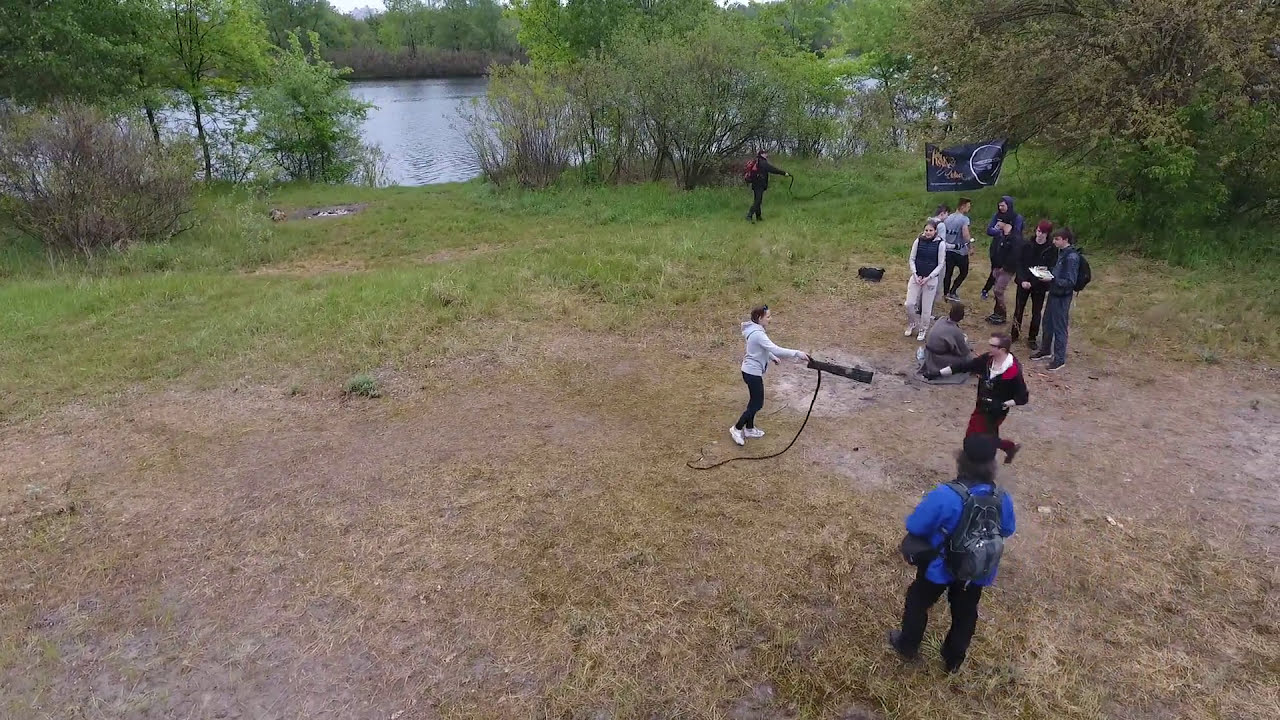This photograph, taken from an elevated perspective, captures a diverse, dynamic ground area with a mix of lush green grass and patches of dried brown grass, indicating frequent foot traffic. The central focus is a group of eight to ten people, some standing and some sitting, engaged in an outdoor activity. Among them, a person stands out wearing a white hoodie, black pants, and light gray shoes, swinging a black tubular object with a cord, possibly a whip.

The foreground of the image is characterized by exposed dirt areas and yellowed grass, suggesting heavy usage, while the background showcases brighter, healthier green grass interspersed with various trees, some fully leafed and others partly shedding. To the far side of the field, a tranquil water body with blue water is visible, bordered by more trees and green grass on the opposite shore.

To the left, a small pond or lake can be seen, surrounded by densely foliaged trees. Positioned near this water body is an unreadable black banner with gold writing, a silver circle, and other silver accents, adding an element of mystery to the scene. The overall setting exudes a lively, yet serene atmosphere of outdoor engagement and natural beauty.